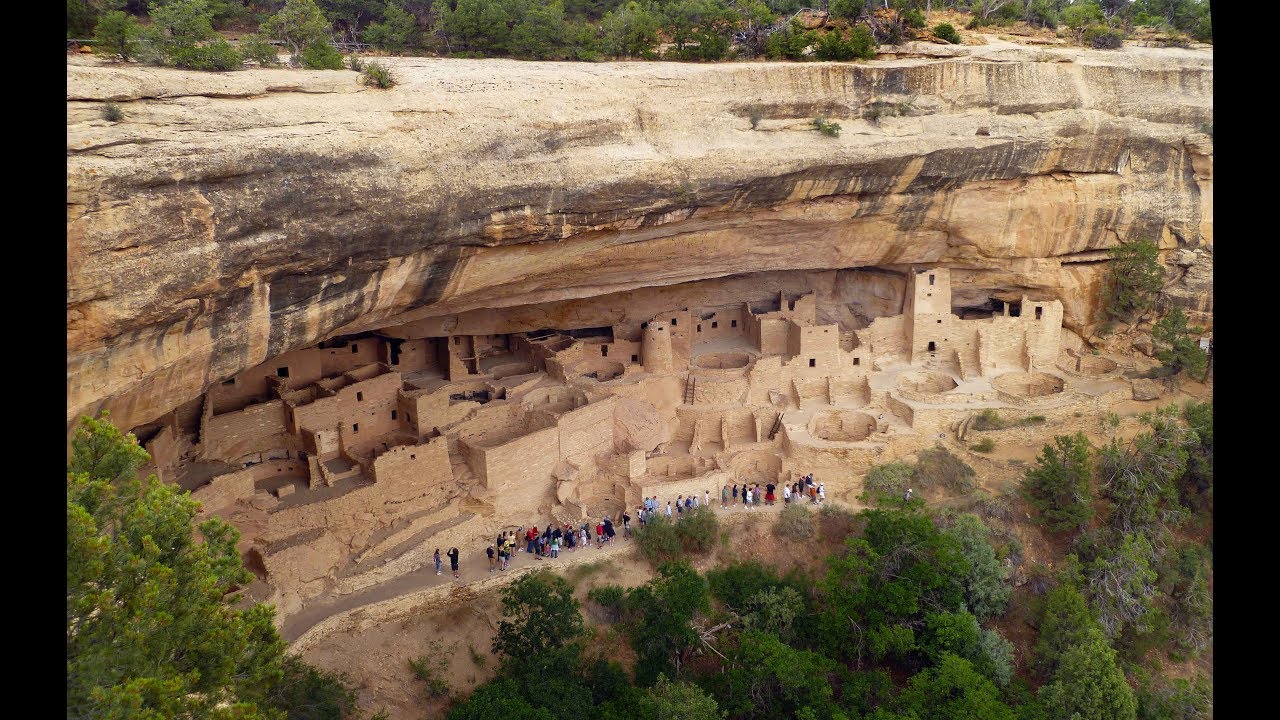The image depicts an archaeological site in the Southwestern United States, showcasing ancient cliff dwellings believed to be constructed by the Pueblo Indians. These clay-like structures are nestled under a massive boulder, with the boulder's overhang acting as a natural roof, providing protection to the city below. The scene captures a tour group of about 20 to 30 people exploring the historic site along a walkway. The cliff above is adorned with green vegetation, and the landscape includes additional trees and greenery along its edge. The entire setting has a desert sand brownish hue, contrasting beautifully with the greenery. The vantage point offers an aerial view of both the archaeological site and the surrounding natural landscape, emphasizing the integration of human habitation within the rugged terrain.